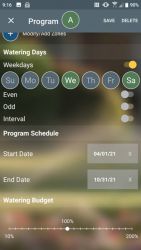**Screenshot of a Mobile Application Interface: Watering Schedule Settings**

The image is a screenshot from a cell phone, displaying the interface of a mobile application likely designed for scheduling watering. The time at the top of the screen reads "9:16", with various icons distributed on both the upper left and right sides. These icons include indicators for Wi-Fi signal strength, cellular connection, and a battery percentage at "98%".

The text within the image is somewhat blurred, making some details harder to decipher, but clear enough to outline the main elements. Below the status bar, there is a gray banner with "Program" written inside, prefixed by an "X" icon, and followed by a green circle containing the letter "A". Next to this, there are options to "Save" or "Delete". A blue circle with a plus sign appears adjacent to some text.

Next, a section labeled "Watering Days" is visible, indicating different days of the week within small circular icons. Days are abbreviated as "S-U-M-O-T-U" for Sunday to Tuesday, presented in gray circles, signifying perhaps inactive or selected days. "W-E" for Wednesday is in a green circle, suggesting an active day. Similarly, "T-H" and "F-R" for Thursday and Friday are in gray circles, and "S-A" for Saturday appears in green.

Underneath, multiple options related to scheduling are listed, such as "Even", "Odd", "Interval", "Program Schedule", "Start Date", "End Date", and "Watering Budget". The budget options are presented as "50%", "100%", and "200%".

On the side, there is a yellow banner titled "Think About", which prompts a series of reflection questions: 

1. What are the images on first glance?
2. What are the objects in their counts?
3. What does the text say?
4. What are the positions of the objects?
5. What subtle details are noticeable?
6. What is the background, and what is the style and color?

The interface design features a mix of gray, green, and blue tones, with a clear structure meant to guide the user through setting up their watering schedule efficiently.